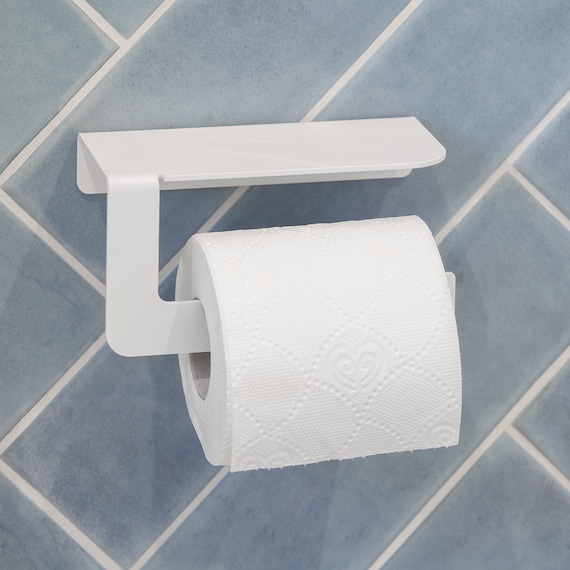The photograph features a partially used roll of toilet paper hanging on a stylized, white metal hook with an L-shaped design and a small shelf on top, suitable for placing an item. The background is a chambray blue tiled wall with rectangular tiles laid diagonally, intersected by clean white grout. The toilet paper, potentially of the AngelSoft brand, displays an embossed pattern featuring diamond shapes, swirls, hearts, and possibly fleur-de-lis motifs. The roll is positioned to hang over and then under, affixed on a holder that is open on the right side, making it easy to slide the paper roll on and off. There are no other objects, colors, artist's marks, or advertisements present in the image, highlighting the simple yet elegant design of the bathroom setting.